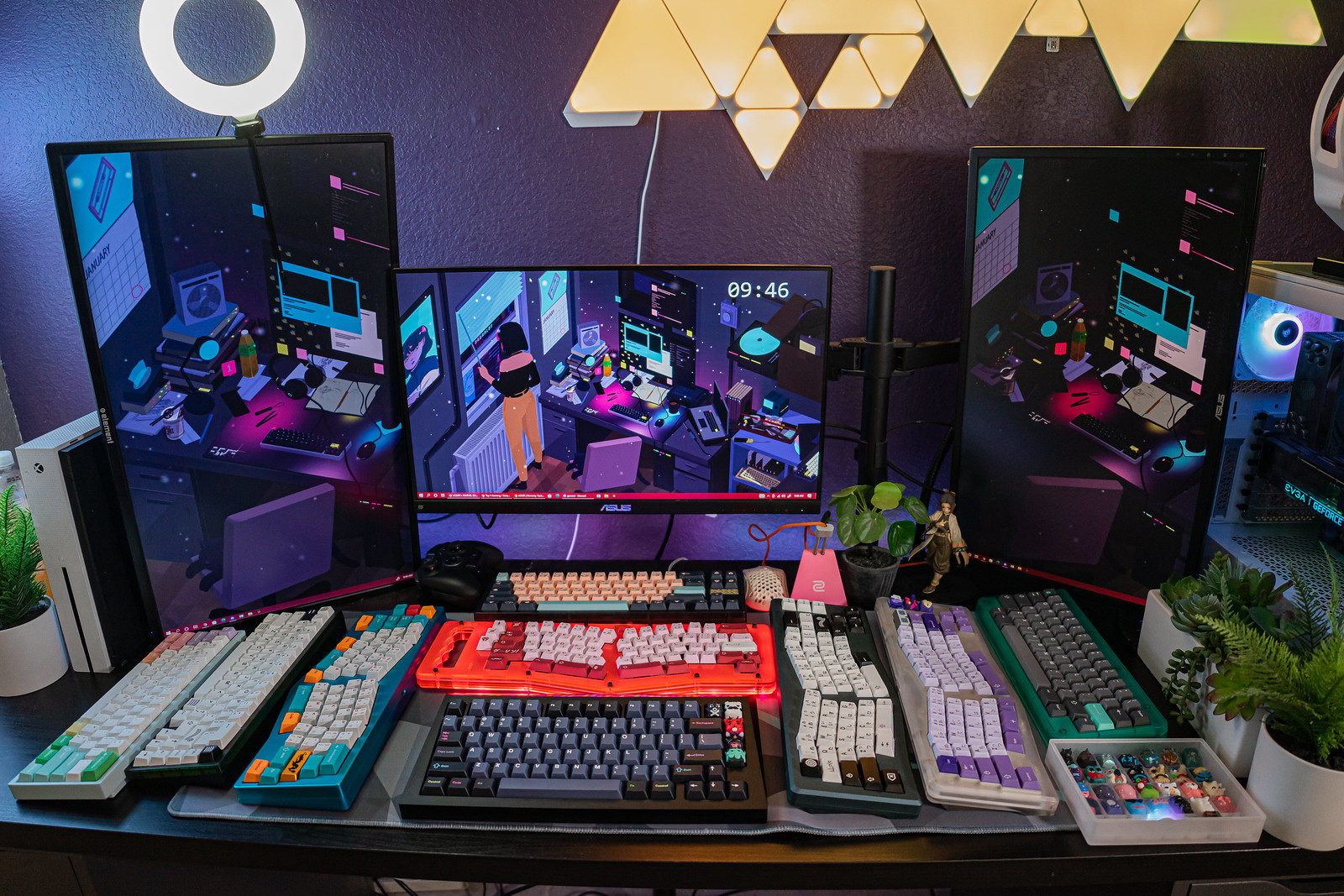The image showcases an elaborate gaming setup on a long desk, designed with a vibrant and retro aesthetic. Central to the setup are three large computer monitors, one vertically oriented on the left with a ring light attached above it, displaying a scene reminiscent of a gaming center with a computer fan. The central monitor features the same retro-themed image, showing a woman looking out a window with bright, colorful sparkles in shades of light blue, teal, and bright purple, and displays the time "9:46." The right vertical monitor mirrors the first one but with a darker background. 

Beneath the monitors, the desk is lined with nine mechanical gaming keyboards in an array of colors: white and green, white and black, teal and orange, white and red, white and pink, black and teal, black and gray, green and white, and purple, white, gray, and green. Each keyboard sits neatly, emphasizing their varied color patterns. Additionally, the setup includes an Xbox lying on its side beside a small green plant, enhancing the organized yet visually stimulating environment meant for a serious gamer or Twitch streamer. The background features a purple wall, further complementing the retro and colorful theme of the setup.